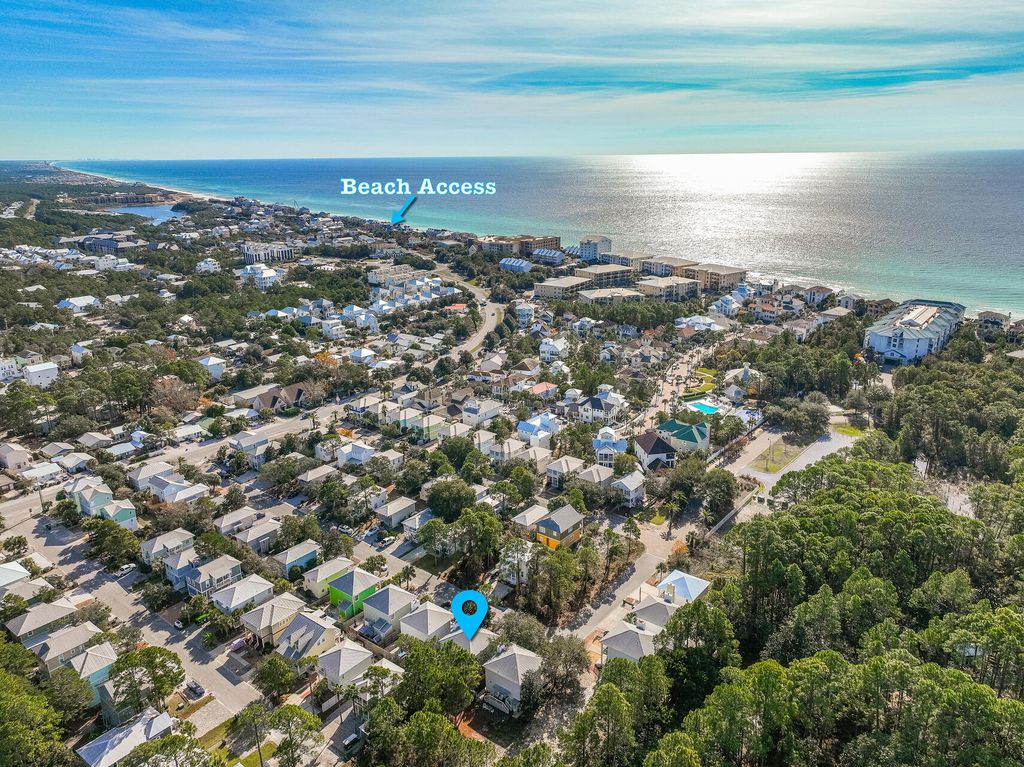A detailed aerial or 3D view showcasing a vibrant residential area nestled near a serene body of water, possibly an ocean or gulf. The image features an array of houses with their roofs in clear view, distributed mostly towards the center-left section. The houses vary in shape, with those in the foreground appearing more similar and tightly knit compared to the others. The top-right quadrant of the picture reveals a calm water body adjacent to a slice of beach, marked by a white text inscription reading "beach access," accompanied by an arrow. Adjacent to the beach is a large rectangular building extending from the shore towards the center of the photo. The upper portion of the image includes a blue sky dotted with clouds adding tranquility to the scene. A road is visible in the lower left center, stretching up towards the upper left corner. The picture is rich in colors, prominently displaying shades of blue, white, black, grey, brown, and abundant green from clusters of trees scattered throughout. Noteworthy is a location icon, colored sky blue, situated towards the bottom of the image, indicating a specific house, suggesting this could be a real estate photograph marking a notable residential property.